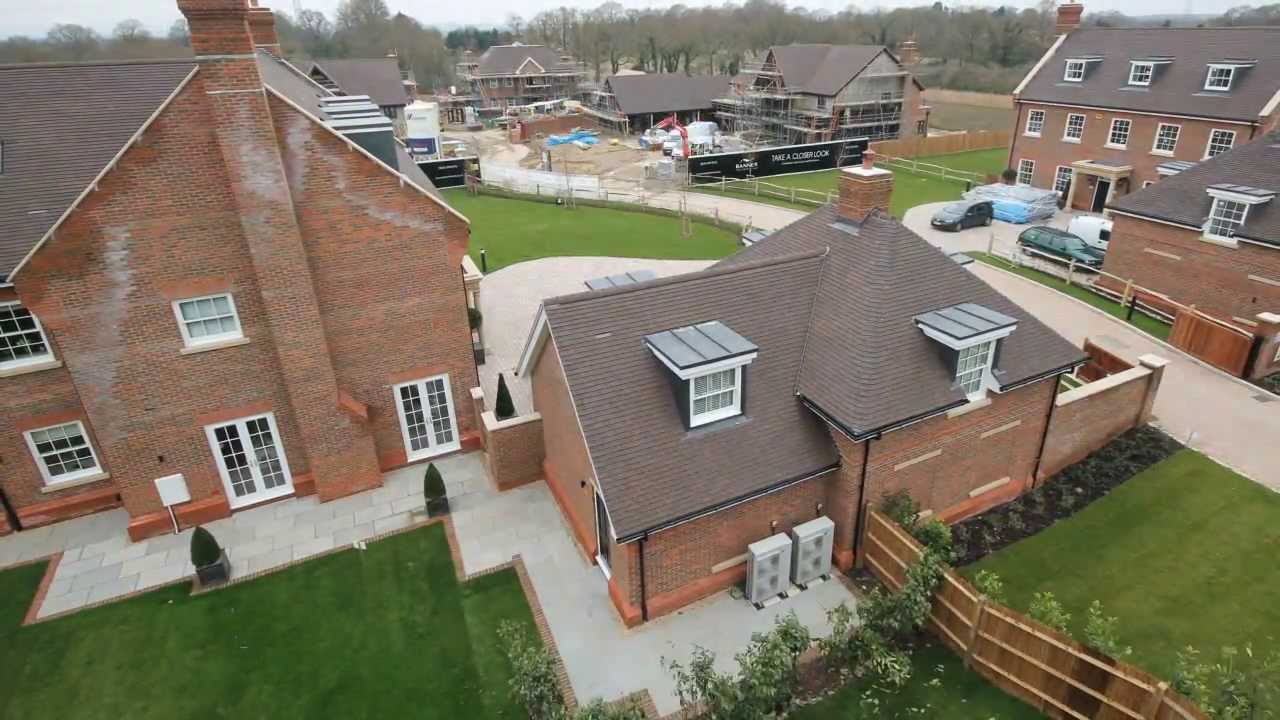The image provides an aerial view of a newly-developed neighborhood featuring seven homes. The primary focus is a red brick house with a dark roof, highlighted by two protruding windows and a chimney. This house features two HVAC units in the backyard, a wooden fence, and a well-maintained lawn. A strip of soil in the backyard indicates recent gardening work. A concrete walkway links this house to an adjacent brick building, likely an apartment complex, which also has protruding roof windows and chimneys, as well as glass doors with multiple panels. In front of this area are two bushy pine-like trees, with another one situated in the upper right.

Surrounding the focal house, the neighborhood consists of red brick homes with dark roofs, white-paned windows, and green lawns enclosed by wooden fences. The neat arrangement of houses includes some still-under-construction, evident by scaffolding and unfinished structures. There are cars parked in front of some houses, suggesting habitation. A road winds through the development, complemented by scattered trees, some appearing dead and indicating a winter season. In the background, construction work is marked by a large banner reading "Take a closer look," drawing attention to an unfinished complex.